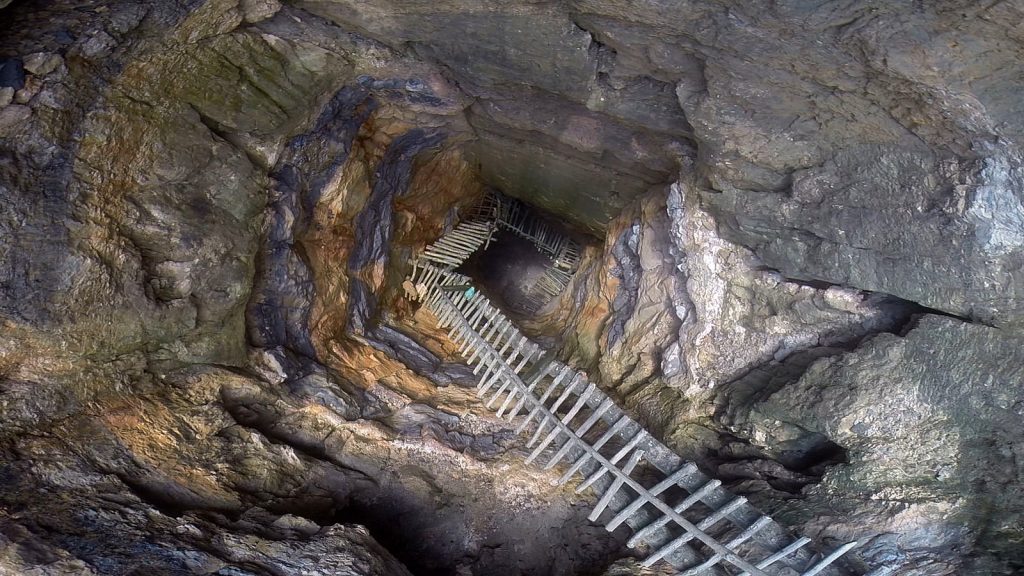This outdoor photograph provides a unique aerial perspective looking down into the mouth of a deep, vertical cave or stone pit. The cave's entrance is surrounded by rugged gray rock, with layers exhibiting hints of yellow and white hues. From this vantage point, it appears as if the viewer is suspended directly over the chasm, potentially captured using a drone camera.

Descending into the cave is a rickety wooden ladder, comprised of weathered, gray boards arranged perpendicular to two parallel supports, resembling an extended series of thick, plus signs. The ladder extends several stories down, creating a precarious spiral as it makes two 90-degree turns along the jagged cave walls. The boards of the ladder appear old and some steps seem loose or broken, adding to the overall feeling of instability.

Daylight illuminates the upper reaches of the cave, creating a stark contrast with the shadowy depths below. The intricate rock formations and the multiple segments of the ladder, possibly remnants of an old mine or quarry, are clearly visible, highlighting the cave’s depth and intricate geology.